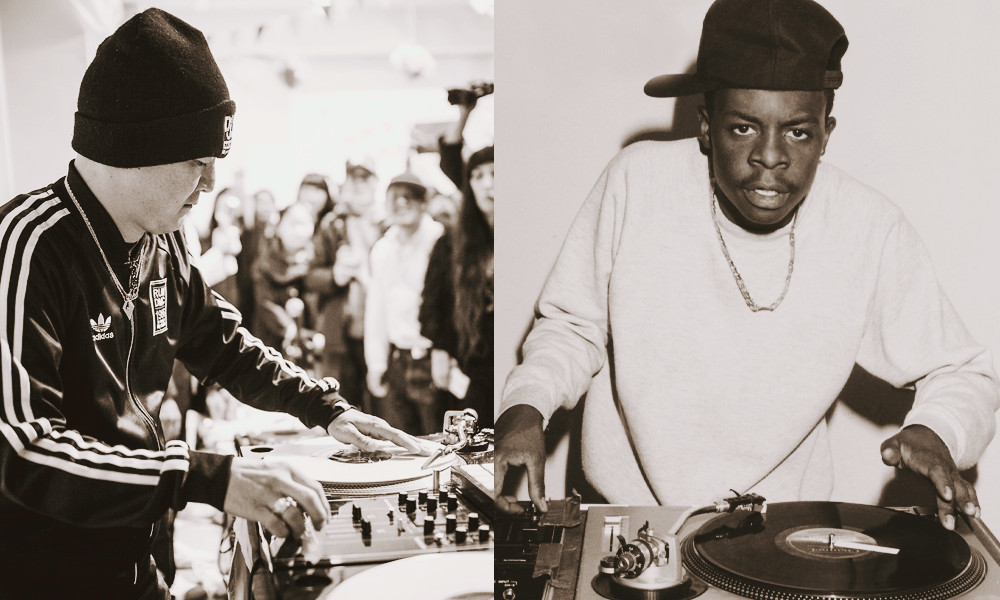In this dual-image illustration, we see two disc jockeys, each captured in dynamic moments. On the left, a man dressed in an Adidas long-sleeve sweatshirt, identifiable by the three stripes on his right shoulder and left arm, is immersed in his craft. His black beanie and the Adidas logo on the right side of his chest, along with some additional text or design on the left, add to his distinct style. Positioned behind his DJ equipment, he is facing the right, engaging an audience in the background who appear to be enjoying the music. On the right, a black man is wearing a cap tilted sideways, a necklace around his neck, and a long sleeve shirt, likely white. He looks directly into the camera with a slightly open mouth, his hands poised over a black disc player. The color palette of both images is rendered in monochromatic black, white, and gray tones, offering a cohesive visual theme focused on the artistry and presence of these two DJs.